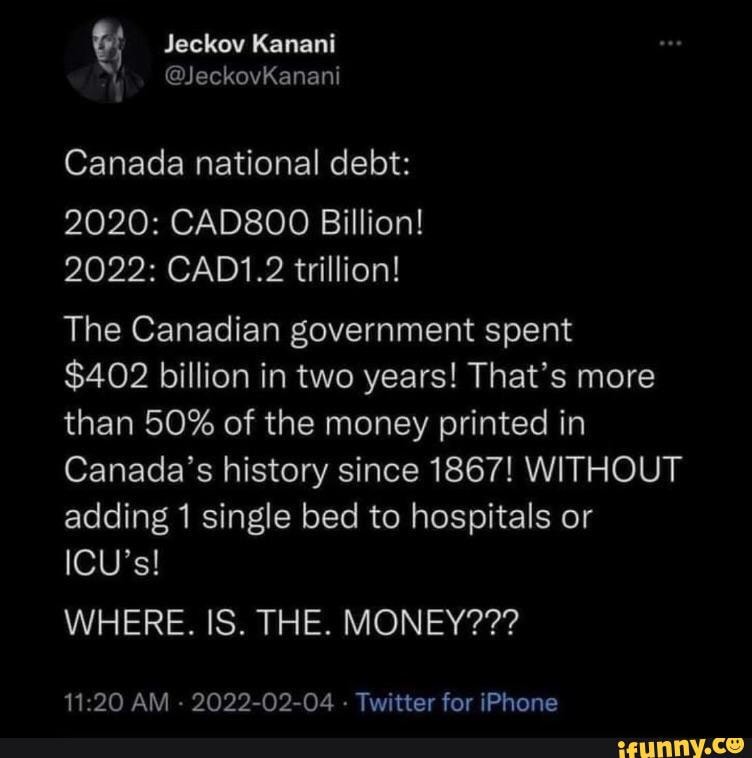This detailed Twitter post includes an evocative black-and-white photograph of a man gazing thoughtfully to the left. The account owner, Chekhov Kanani (@ChekhovKanani), is identified in the upper left-hand corner by their profile picture and handle. The post, timestamped at 11:20 a.m. on February 4th, 2022, from Twitter for iPhone, addresses the sudden increase in Canada's national debt. The text highlights that the debt rose from $800 billion in 2020 to $1.2 trillion in 2022, noting that the Canadian government spent $202 billion over two years. The user points out that this amount represents over 50% of the money printed in Canada's history since 1867, and criticizes that the expenditure did not result in additional hospital beds or ICU capacity. The post culminates in a dramatic, all-caps query, "WHERE. IS. THE. MONEY???" In the lower right-hand corner, a yellow annotation reads, "iPhone, not you."